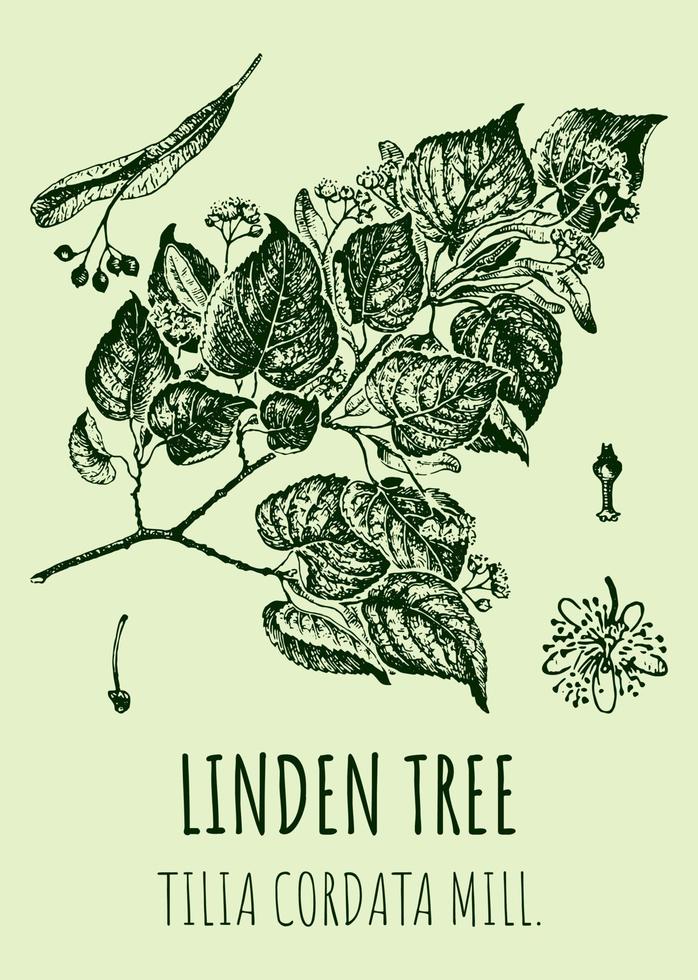This black pen illustration, set against a pale yellow-green background, intricately depicts a small branch of a plant, reminiscent of a twig, showing off its detailed structure. The main branch extends to reveal multiple smaller branches, each adorned with varying numbers of leaves ranging from three to six. These leaves are distinctively shaped like upside-down hearts, with pronounced veining detail that adds to the botanical precision of the sketch.

Interspersed among the leaves are delicate flowers and seed pods. The flowers, each with five petals, are depicted with fuzzy stamens, adding a realistic texture to the illustration. Additionally, there are slender, elongated seed pods and tiny twigs bearing clusters of berries, enriching the plant's portrayal.

Beneath this elaborate depiction, the text “LONDON TREE TILIA CORDATA MULL” is inscribed in black, identifying the illustrated plant as the small-leaved lime, also known as Tilia cordata.